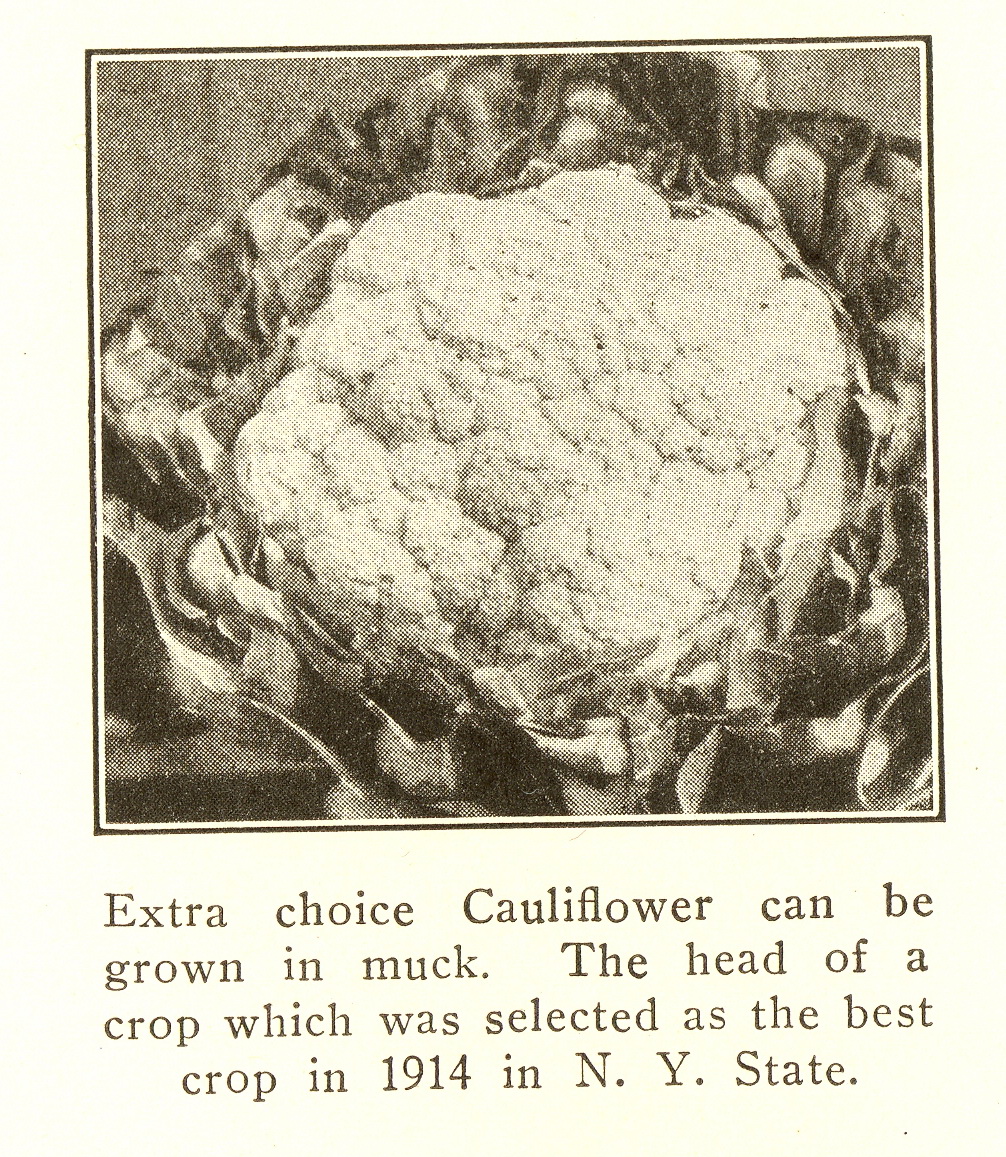The image depicts an old, tan, dot-matrix printed newspaper or magazine snippet, centered around a grainy black and white photograph of a large head of cauliflower with leaves surrounding it, possibly set on a table. The photograph occupies the top portion of the image and is framed in black and white. Below the picture, the aged, distressed paper features black text that reads: "Extra-choice cauliflower can be grown in muck, the head of a crop which was selected as the best crop in 1914 in New York State." The entire image exudes a vintage, historical feel, accentuated by random dots and marks indicative of its age.